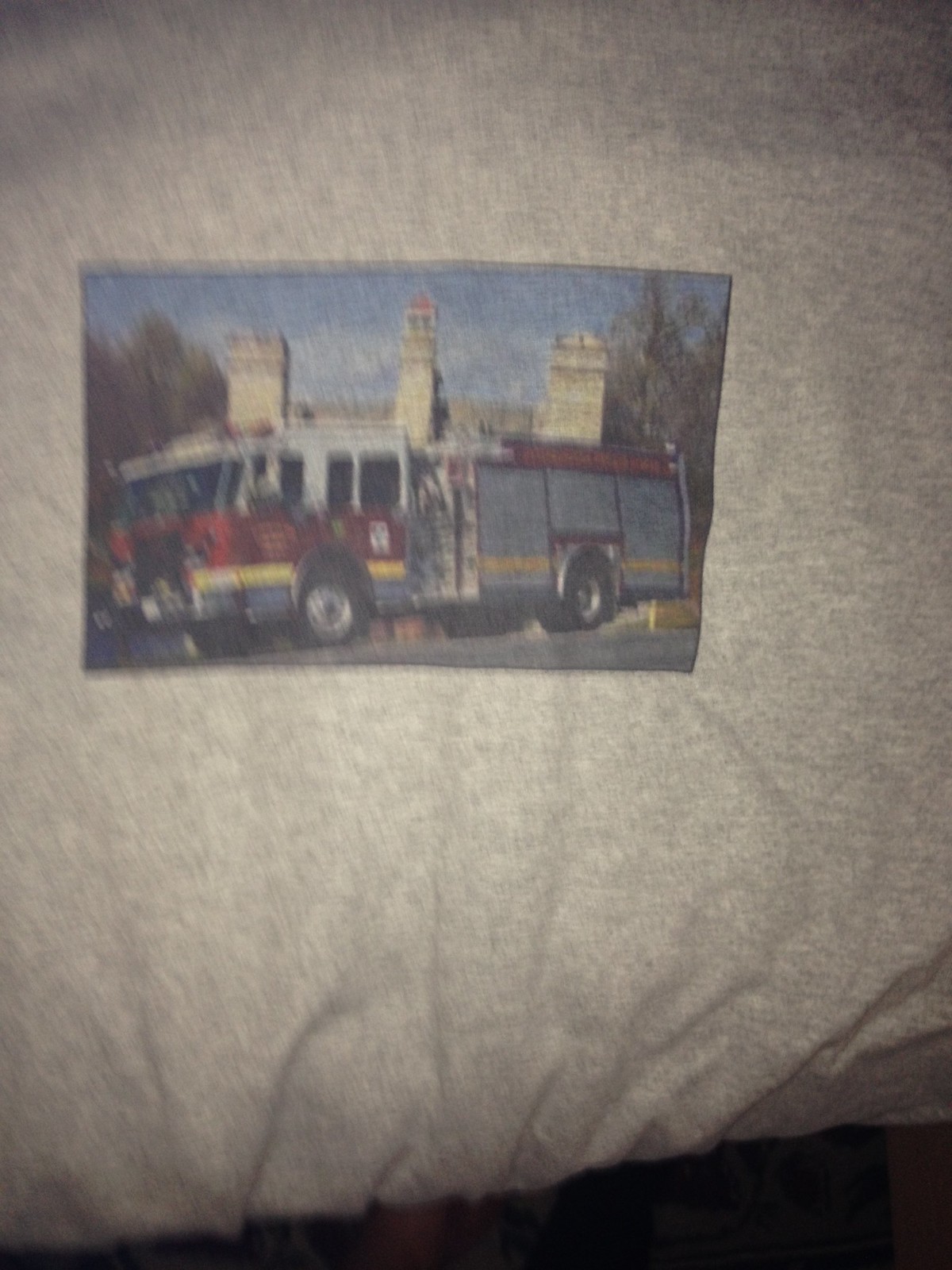This blurry photograph captures a gray garment that could either be a t-shirt or a sweatshirt. At the center, a graphic depicts a fire truck in motion, traveling from right to left in a side profile. The fire truck features red, white, and yellow horizontal bars along its top, and its rear showcases small garage-like doors for accessing hose connections. The truck's tires are black. In the blurry background, a structure resembling a church is visible, though there is no indication of fire. Due to the blurriness, any text on the fire truck is illegible.